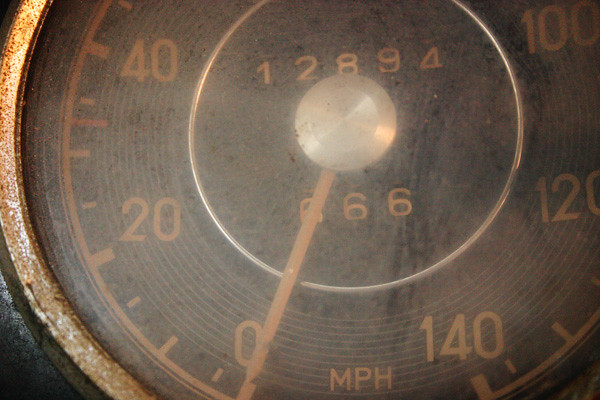This photograph captures a classic automobile dashboard, focusing on the odometer and speedometer gauges. The odometer, centered prominently, has a dark brown background with pale tan numbers. The primary odometer reading shows 12,894 miles, with a smaller secondary reading displaying 0666, part of which is obscured by the needle. The gauge’s crescent-shaped needle rests at zero, indicating acceleration is halted.

Surrounding the odometer, a slightly corroded copper rim adds a vintage aesthetic, contrasting against the enclosing black metal structure. Above the odometer is a round, steel-framed speedometer. The speedometer dial progresses from 0 to 140 mph in 20-mile increments, with smaller ticks marking intermediate speeds. The overall condition and design suggest a vehicle from a bygone era, characterized by its utilitarian yet elegant instrumentation.